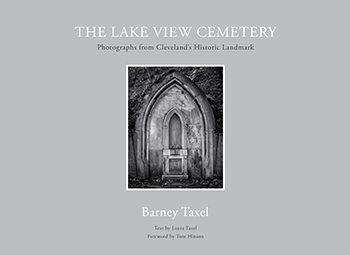The image appears to be the cover of a book or CD case set against a solid gray background. In the center, there is a squarish, charcoal gray sketch design bordered with a white outline. The focal point is a smaller doorway-like shape within a larger tapered, leafy or iron-shaped design, possibly indicating an architectural feature of a cemetery or church building.

At the top of the cover, prominently displayed in all-capital letters with white text, it reads "The Lakeview Cemetery." Beneath this, in smaller black text, it states "Photographs from Cleveland’s Historic Landmark."

Below the central image, in white text, the name "Barney Taxel" is prominently featured. Underneath this name, there are two lines of black text, which are too small to discern clearly, possibly indicating credits or additional information about the contributions to the publication.

Overall, the cover design, with its meticulous details and contextual clues, strongly suggests it pertains to Lakeview Cemetery in Cleveland, Ohio, likely showcasing a collection of photographs from this historic site.